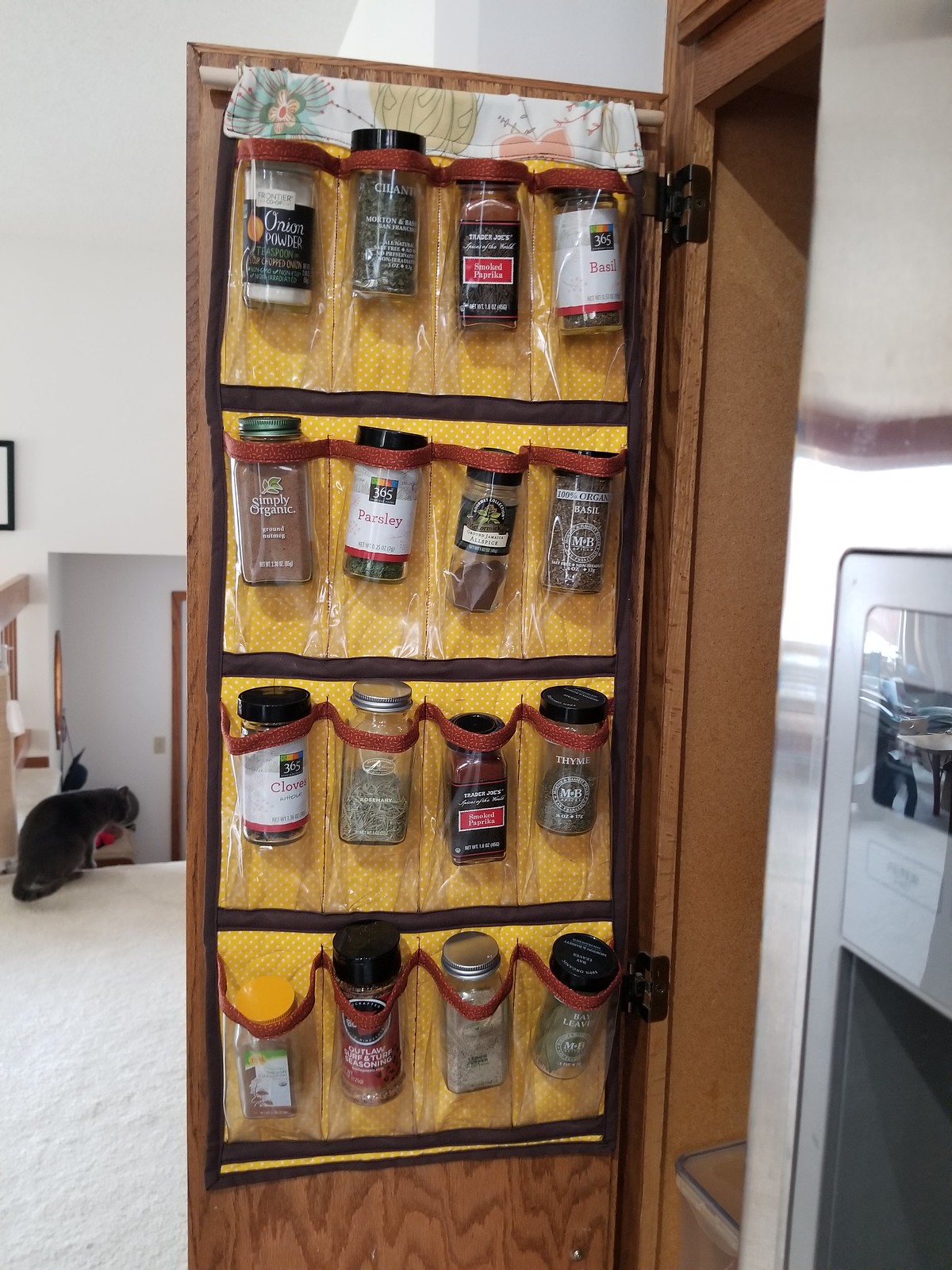This image captures the open door of a pantry in a kitchen, prominently featuring a spice rack that hangs from a dowel at the top of the pantry door. The spice rack consists of clear plastic pouches against a yellow polka-dotted background, displaying an array of 16 spice bottles. Among the identifiable spices are red pepper flakes, thyme, parsley, basil, cinnamon, onion powder, paprika, a second bottle of basil, and bay leaves. To the right of the door, the edge of a refrigerator with an ice dispenser is visible. The scene further includes a grey cat, likely grooming itself, sitting on the carpeted floor just inside the pantry. Additionally, part of the house, including what appears to be the front door and a picture frame intruding from the left side, is faintly discernible in the background. The overall setting implies a well-organized kitchen space with a thoughtful design.